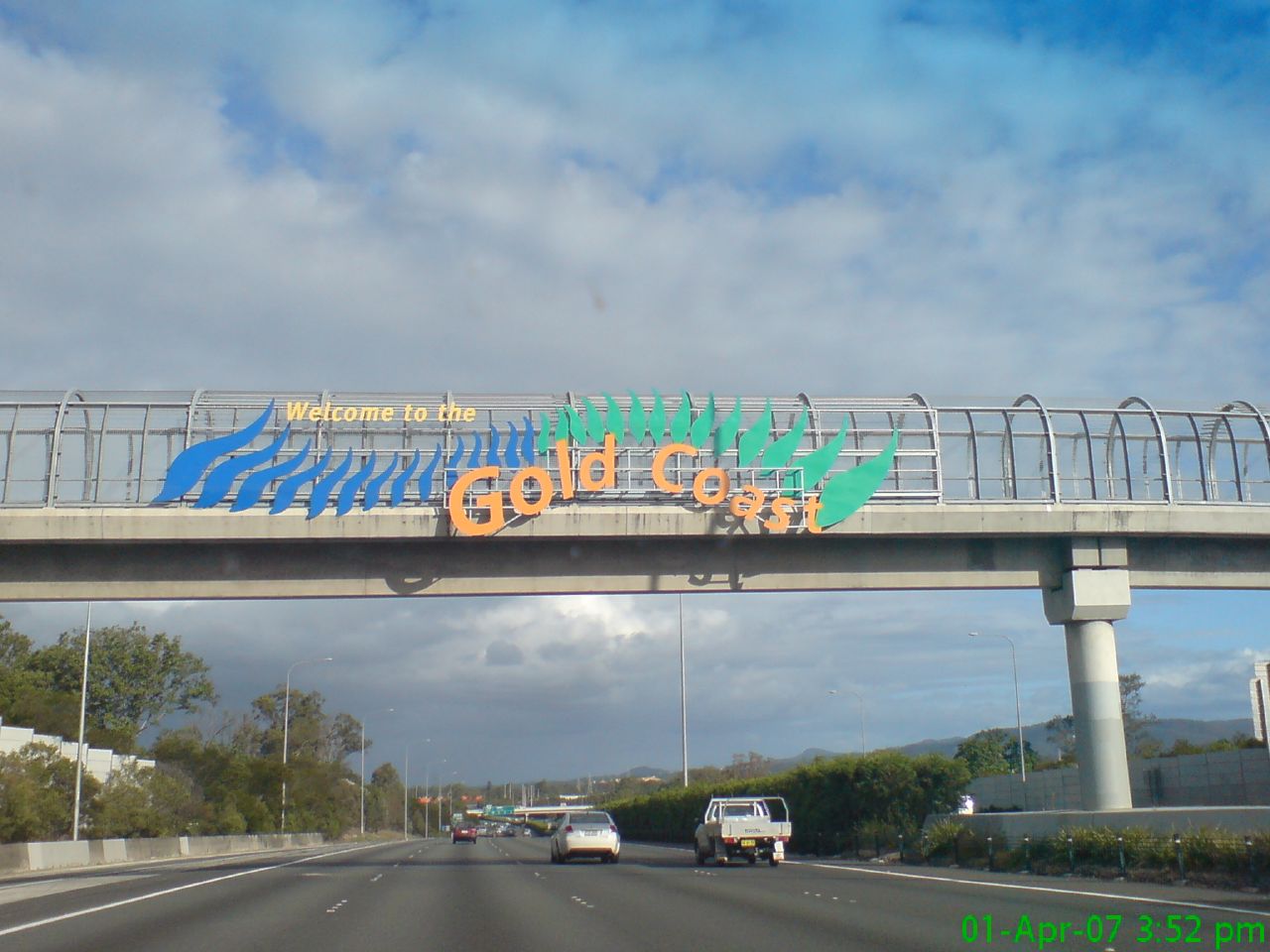The photograph captures a vibrant daytime scene along a four-lane highway, viewed from behind the cars as they travel away from the viewer. Dominating the center of the image is a concrete pedestrian overpass equipped with metal barriers acting as a protective cage. The overpass prominently displays a welcoming sign in a wave pattern with "welcome to the" in yellow and "Gold Coast" in orange, flanked above by blue and green wavy lines, adding a touch of artistic flair.

Above the highway, the sky transitions from being partly cloudy at the horizon to a clearer, bright blue as it extends upward and to the right. On the right-hand side of the highway, you can see concrete barriers and a scattering of shrubbery. Tall streetlight posts line both sides of the road, and distant trees dot the landscape on the far side. Off in the distance, more cars can be seen further down the highway amid green roadsides.

In the lower right-hand corner of the image, there is a timestamp reading "01 April 07, 3:52 PM" in green lettering. The meticulous details of the scene evoke an ordinary yet serene moment on a well-traveled road, framed by the welcoming message of the Gold Coast.